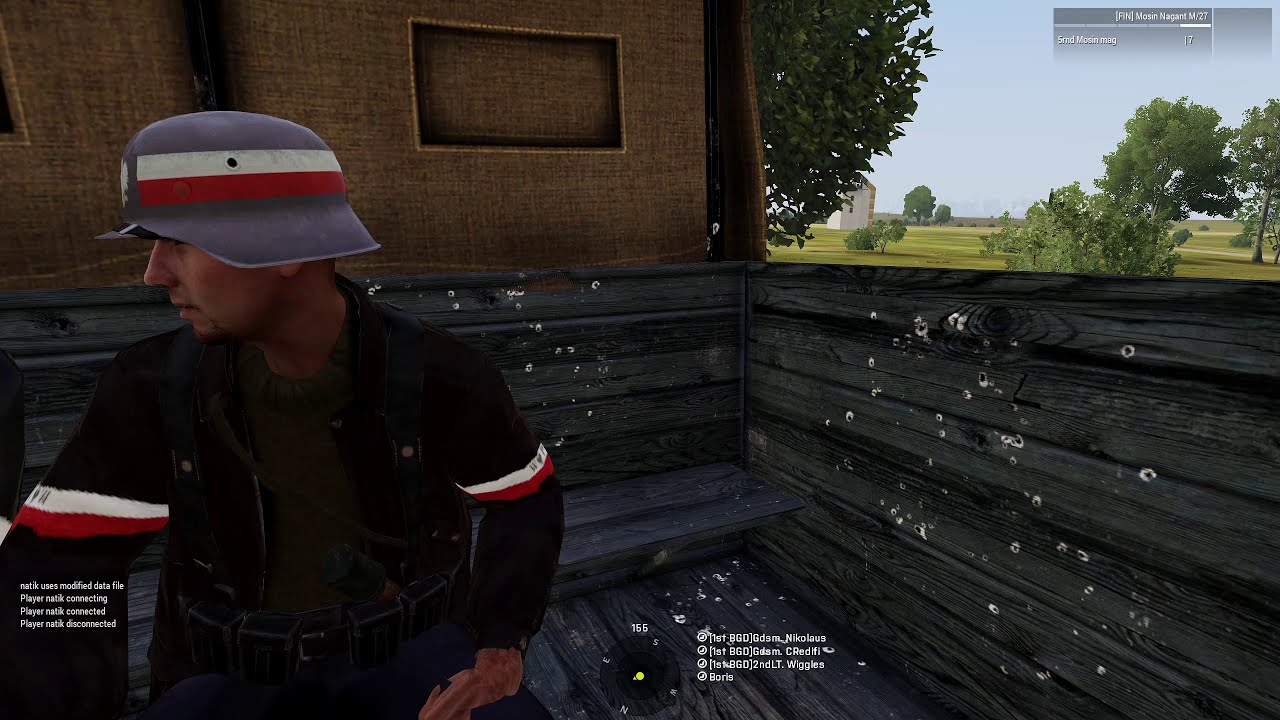The image appears to be a screenshot from a first-person video game, showcasing a cartoon-like character within a natural, rustic setting. The character, who has notable alterations such as an odd-looking left hand, is dressed in a dark blue smock featuring white and red stripes, complemented by a light blue helmet adorned with the same stripe pattern. The character's peach-colored skin contrasts with the wooden textures of what seems to be a truck bed they are sitting in, taking up the lower portion of the image.

Behind the character, the landscape includes expansive fields, trees, and an old farm building that appears white and brown, set against a backdrop of green grass and a blue sky. The top right of the image reveals more of this pastoral scenery, including bushes and open fields, emphasizing the outdoor and likely daytime setting. Superimposed text, indicative of in-game notifications, is present but difficult to read, blending into the gray and black elements of the background.